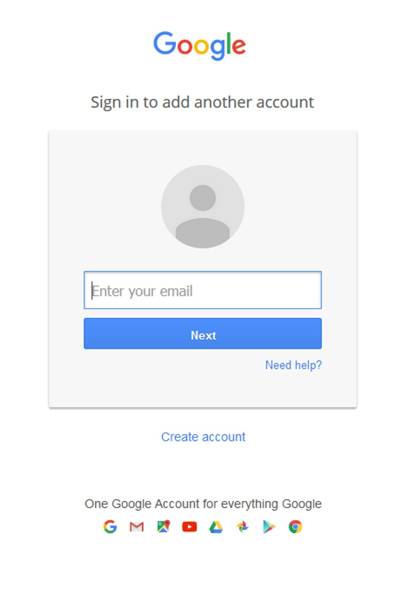The image depicts a Google sign-in page designed for adding an additional account. The layout lacks a defined boundary, encapsulating only a partial frame. 

At the top center of the page, "Google" is prominently displayed in its signature multicolored letters: blue, red, yellow, and green, set against a clean white background. 

Beneath the Google logo, dark gray text instructs users to "Sign in to add another account." This section is followed by a pale gray rectangular area. Positioned at the top center of this area is a circular user profile icon, featuring a light gray background with a darker gray, generic head-and-shoulders silhouette representing the standard profile image.

Below the icon, two interactive horizontal text boxes are present. The first box is white with a bright blue border, and the cursor is located at the far left inside it. This box contains the placeholder text "Enter your email" in gray. Directly beneath this, there is a vibrant blue rectangular button with the word "Next" boldly displayed in white, centered within it. 

To the right of the "Next" button, the text "Need help?" appears in bright blue. Just below the pale gray section, another clickable option "Create account" is highlighted in bright blue.

At the very bottom, gray text states, "One Google Account for everything Google," followed by a row of colorful icons representing various Google services: Google, Gmail, Google Maps, YouTube, Google Drive, Photos, an unidentified service, and Chrome.